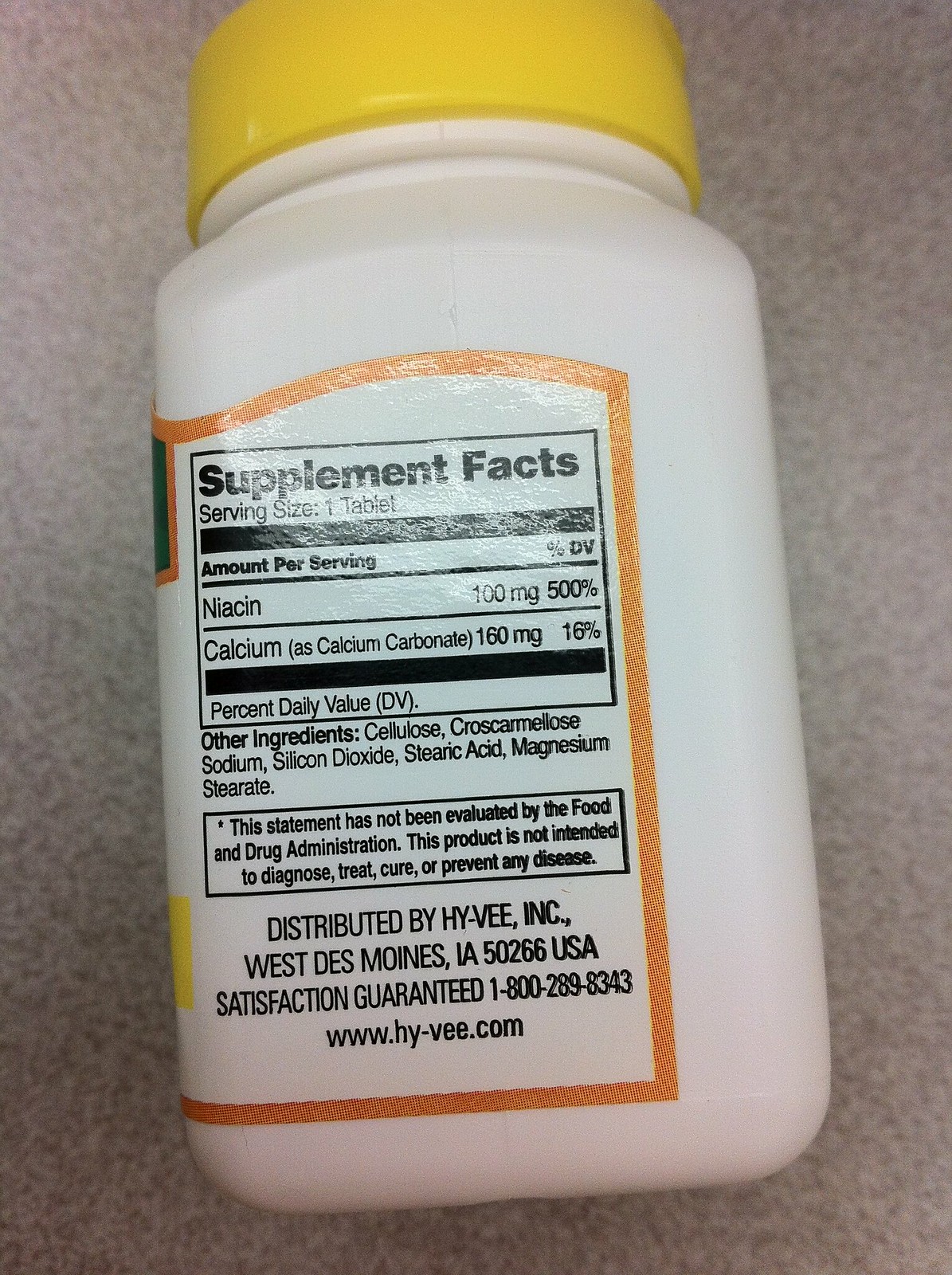In this image, there's a white plastic bottle of pills or supplements with a bright yellow cap. The bottle is short and has four corners, with a white label partially wrapped around it. The label features an orange border and details the supplement facts. It reads "Supplement Facts" at the top, followed by "Serving Size 1 Tablet." Below that, there is a black bar separating further information, including "Amount Per Serving," which lists "Niacin 100mg (500% DV)" and "Calcium 160mg (16% DV)." Additional sections mention other ingredients and daily values. Towards the bottom of the label, there's a block of text indicating the distributor: "HY-VEE Inc., West Des Moines, Iowa, 50266 USA," along with the phrases "Satisfaction Guaranteed," a customer service phone number (1-800-289-8343), and the website (www.hy-vee.com). The bottle is set against a gray background, providing a clear view of the detailed label and bright yellow cap.